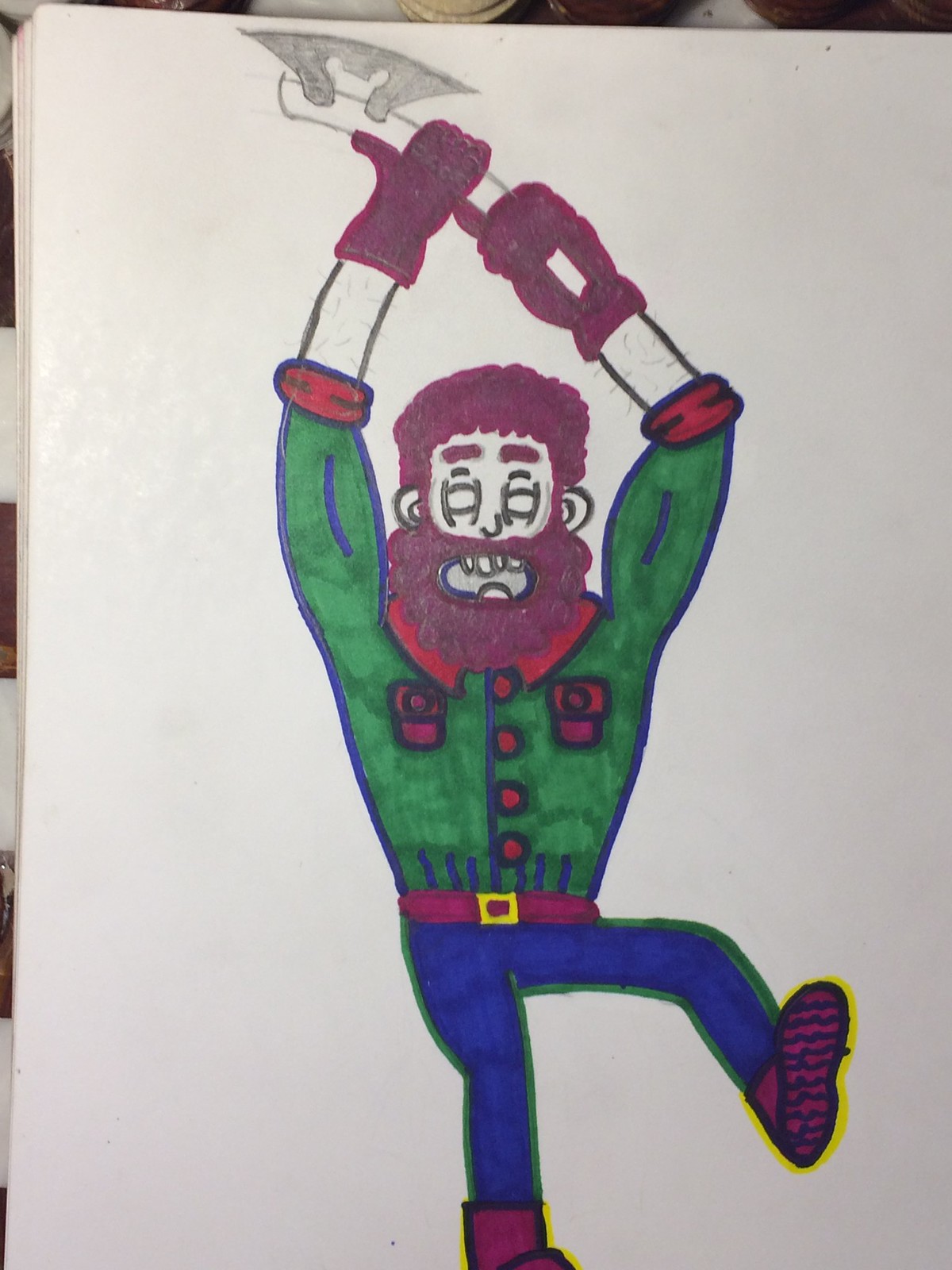This image is a vividly colorful marker drawing on a white piece of paper, depicting a comic-style lumberjack in dynamic motion. The lumberjack is dressed in a green long-sleeve shirt with rolled-up sleeves revealing red cuffs. The shirt features red buttons, a red collar, and red pockets on either side of the chest. He wears a pink belt with a gold square buckle over blue jeans. His right leg is lifted and bent at the knee, showcasing the sole of his red work boots, which have black details and are outlined in yellow. His left leg is slightly bent, providing a sense of action. The lumberjack has burgundy hair that blends into a beard, and his mouth is open, displaying his upper teeth and a pink tongue. His arms are raised above his head in a triangular formation, wielding a white axe with a black head as though preparing to chop. Red gloves cover his hands, and his muscular forearms are highlighted with black lines representing hair. Overall, the drawing captures the energetic and robust essence of a lumberjack in mid-swing, ready for action.